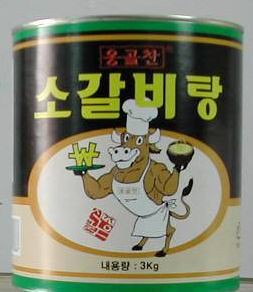This vibrant color photograph features a close-up of a green can, set against a backdrop that transitions from light grey at the top to darker grey at the bottom. The can's edges are silvery, which frames an inner black background adorned with red and yellow Chinese symbols.

At the center of the can's design is a charming cartoon depiction of a cow standing on its hind legs. The cow, with medium brown fur, is dressed as a chef, sporting a white chef's cap and a white apron tied around its neck and waist. 

In its left arm, positioned on the right side of the image, the cow holds a black bowl containing a yellow substance. In the other arm, it holds a tray featuring a Chinese character. Below this illustration, there is a red barcode-like element. The weight indication "3 kilograms" is inscribed in black text near the bottom of the can.